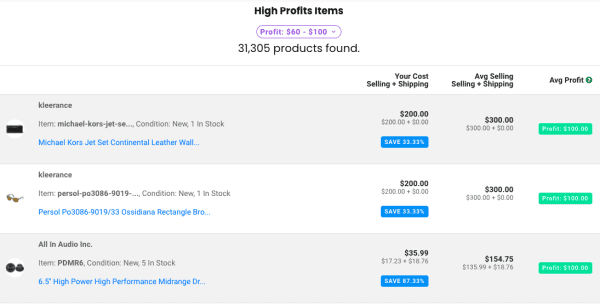The image is a computer screenshot predominantly featuring a white background with black and blue text, arranged horizontally. 

At the top, there is a title in black text: "High Profit Items." Below it, in a purple oval, blue text reads: "Profit $60 to $100." Centered beneath this is black text stating, "31,305 products found."

The main content comprises lists of products organized in gray bars. The first bar mentions a misspelled "clearance" item (spelled with a K) and describes:
1. **Item**: Michael Kors Jet Set Continental Leather Wallet
   - **Your Cost (Selling & Shipping)**: $200
   - **Average Selling & Shipping**: $300
   - **Average Profit**: $100

The next section includes:
2. **Clearance Item**: An unspecified "personal" condition, marked as "new," with only one item in stock. Details mention "Ocidiana Rectangle VRO," which appears to be a type of sunglasses.
   - **Your Cost (Shipping & Selling)**: $200
   - **Average Selling & Shipping**: $300
   - **Average Profit**: $100

The final product listed is:
3. **Item**: All-in-Audio Ink, 6.5-inch High Power High Performance Mid-Range (partially obscured text)
   - **Visual**: Two black circular objects, likely components of the audio equipment
   - **Your Cost**: $35.99
   - **Average Selling & Shipping**: $154.75
   - **Average Profit**: The amount is unreadable in the screenshot.

Overall, the image outlines high-profit items and provides specific details about costs, selling prices, and profit margins for featured products.